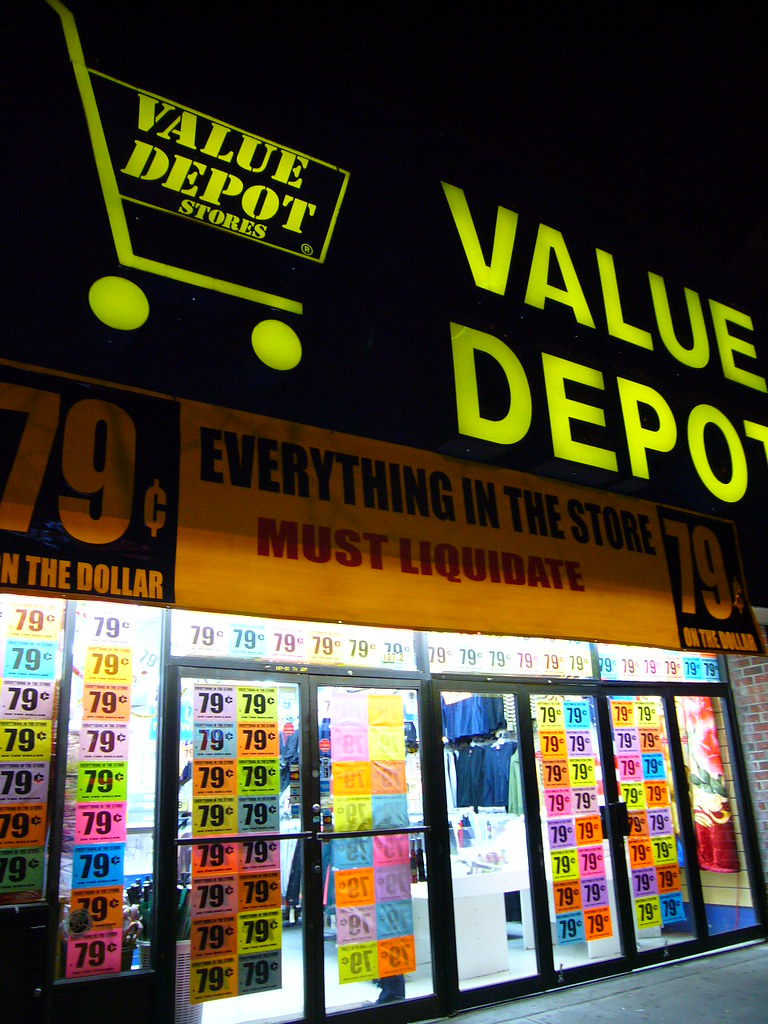This nighttime image captures the exterior of a city building, specifically the storefront of "Value Depot." Dominating the scene is a vibrant neon yellow store sign that illuminates the surroundings. Below this bright sign hangs a large orange and black banner proclaiming "Everything in the store, 79 cents on the dollar." The store's windows and doors are plastered with numerous colorful stickers, all prominently displaying the 79-cent sale, in shades of yellow, pink, blue, orange, and purple. The interior of the store, visible through the glass, is well-lit and reveals rows of hanging clothing, indicating that the store is open and bustling with activity.